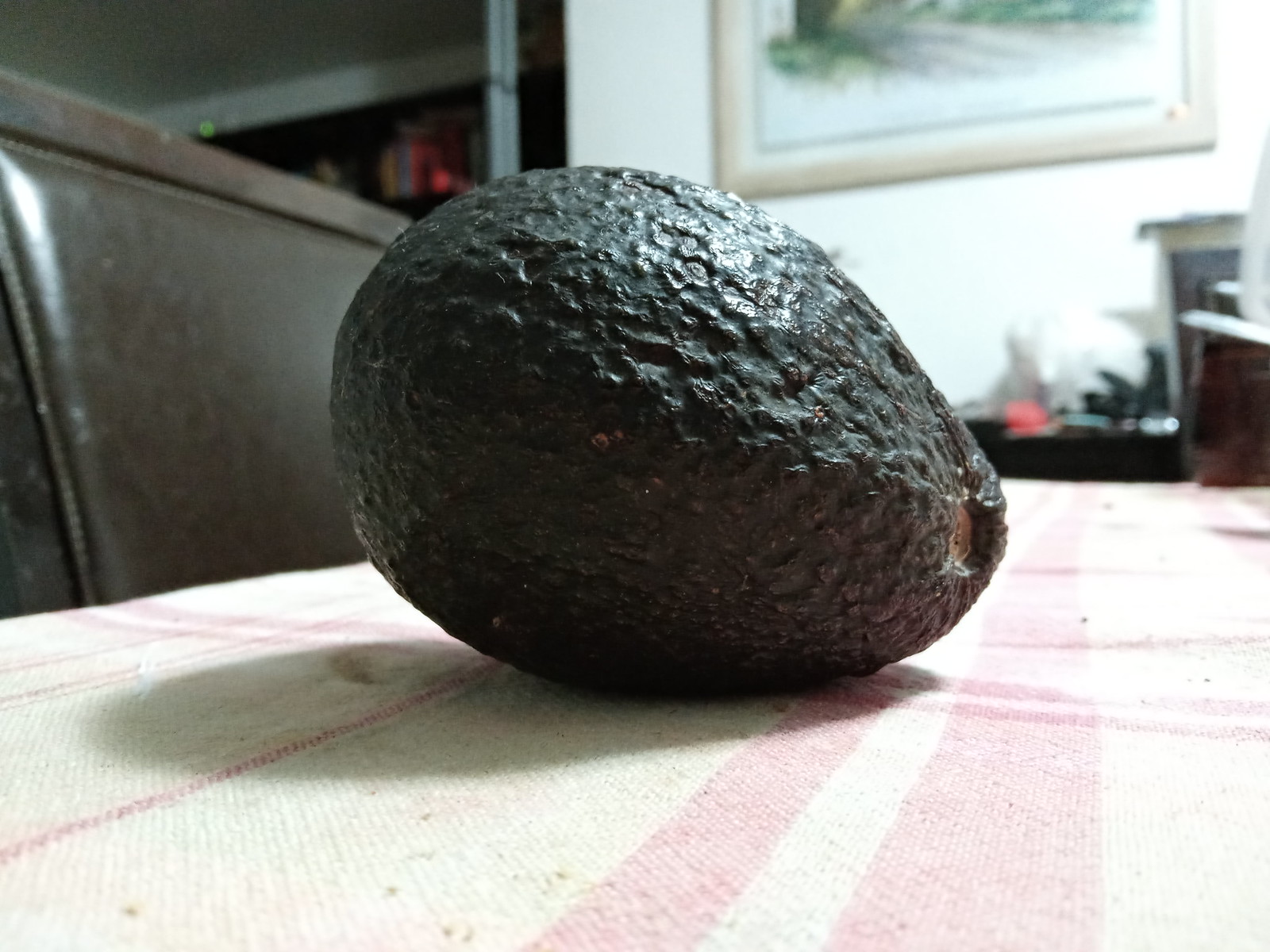This detailed photograph showcases a close-up of a ripe Haas avocado resting on a table covered by a white tablecloth with subtle pale pink or lighter gray lines. The dark green, knobbly-skinned avocado, which still bears the small round button from the removed stem, is the focal point of the image. Situated on the left side of the photo is a brown leather banquette, suggesting the setting could be a restaurant booth or a cozy home corner. In the background, there's a white wall adorned with a framed painting, which has a mix of green and gray hues and is set in a brown or white frame. Below the painting, there appears to be a somewhat cluttered desk or table filled with various objects, adding depth and context to the scene. Shadows cast by the avocado hint at the light's angle, enhancing the texture and detail of both the fruit and its surroundings.